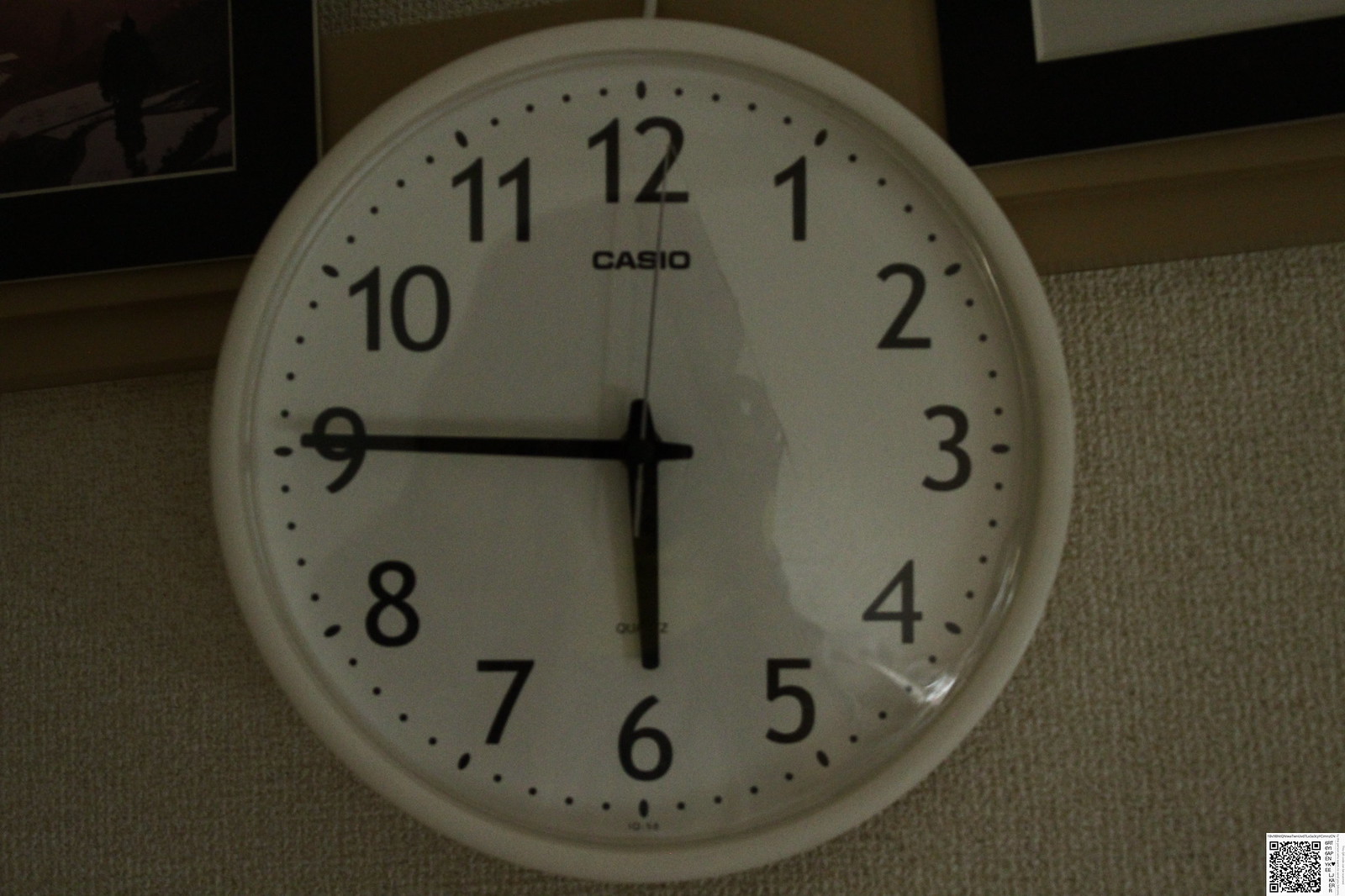The image features a centrally positioned, circular wall clock with a white face. The clock displays black numeric numbering from 1 to 12 and has black hands indicating the time as 5:45. The clock is mounted on a wall, which serves as the background. The wall hosts two dark brown picture frames situated in the top left and right corners relative to the clock. The lower portion of the wall has a gray, almost cotton-like texture, blending shades of white and gray. A light tan or light brown border runs along the top of the wall. Additionally, the reflective surface of the clock face captures a faint image of the person taking the photograph.